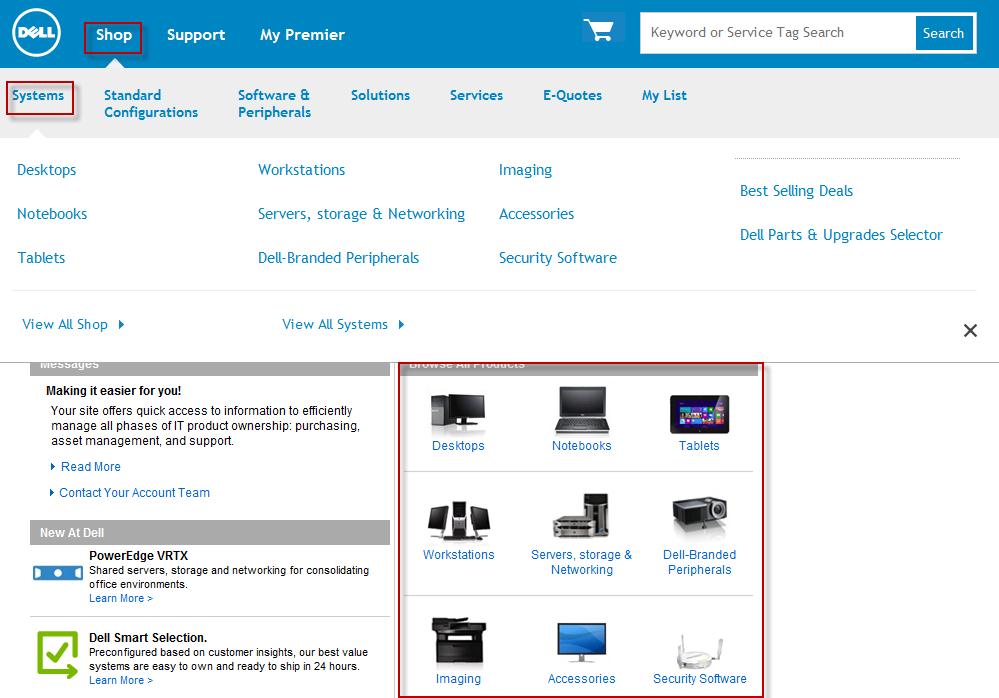The webpage features a prominent blue banner at the top, showcasing a white circle with the Dell logo in white text. Adjacent to the logo are navigation options: "Shop," "Support," "My Premier," a white shopping cart icon, and a search button. Below the banner lies a menu with blue text, offering categories such as "Systems" (highlighted within a red square), "Standard Configurations," "Software," "Solutions," "Services," "E-Quotes," and "My List."

The page is organized into three horizontal rows of blue text on a white background. The first row lists "Desktops," "Workstations," and "Imaging." The second row includes "Notebooks," "Servers," "Storage," "Networking," and "Accessories." The third row mentions "Tablets," "Dell-branded Peripherals," "Security Software," and options to "View All Shop" and "View All Systems."

Towards the bottom left, there are three paragraphs in black text, but the font size is too small to read clearly. On the right side, there are images showcasing various product categories: Desktops, Notebooks, Tablets, Dell-branded Peripherals, Security Software, Accessories, Imaging, Servers, Networking, and Workstations. The Workstations section is highlighted with a red-outlined square.